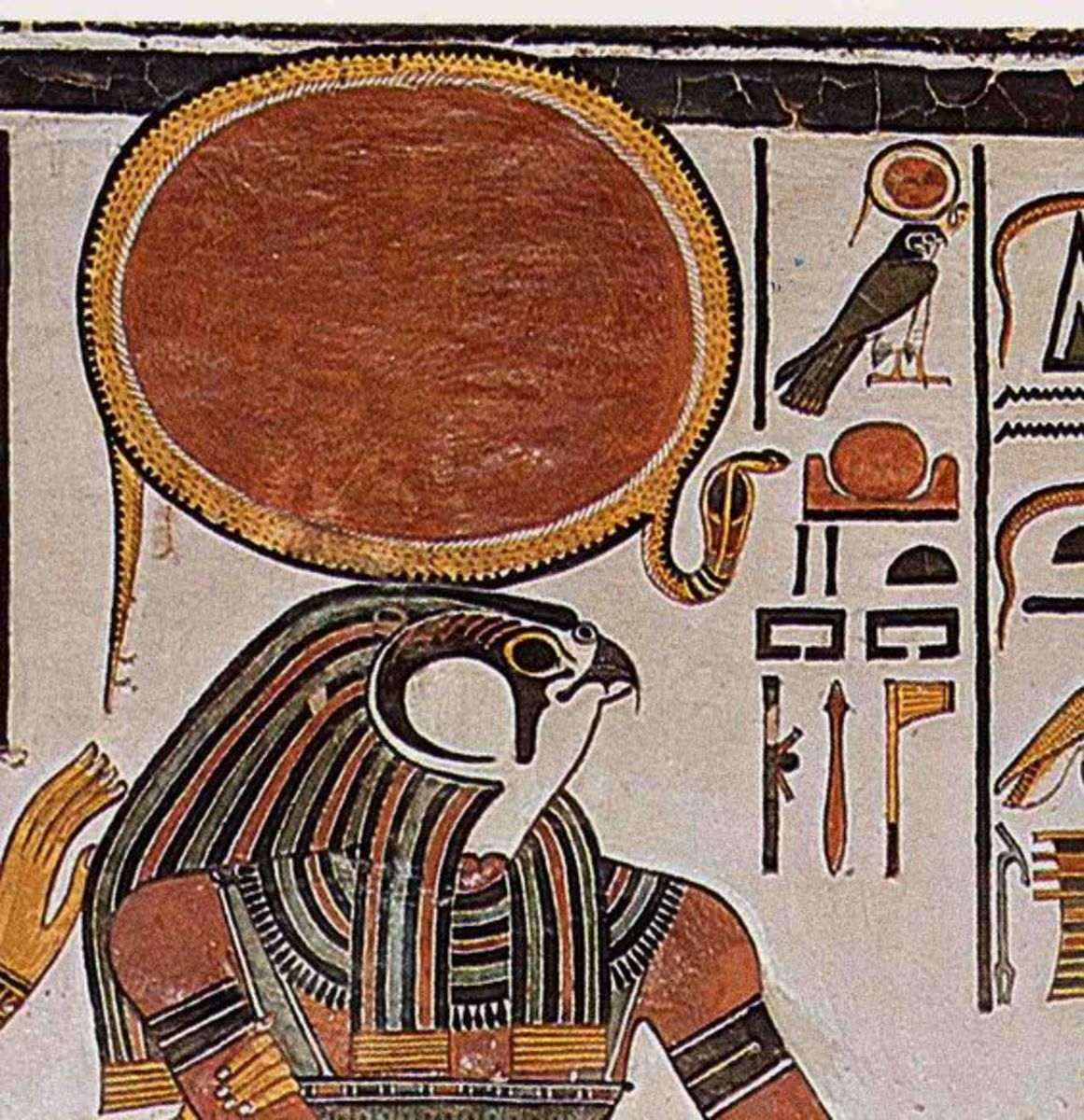The painting depicts an ancient Egyptian artwork featuring the god Ra, identifiable by his falcon or hawk head adorned with dark brown and golden hues, and wearing distinguished royal attire that includes scarves and regal sashes. The image is detailed with intricate hieroglyphics to the right, though some are faded or cut off. Dominating the bottom portion of the image, the god Ra stands prominently, while a cobra, artistically coiled around a large circle, hovers just above him. This circle possibly signifies something significant like the sun. The artwork is well-preserved overall, with only minor cracking and wear, and evokes a sense of both ancient cave art and detailed tapestry.